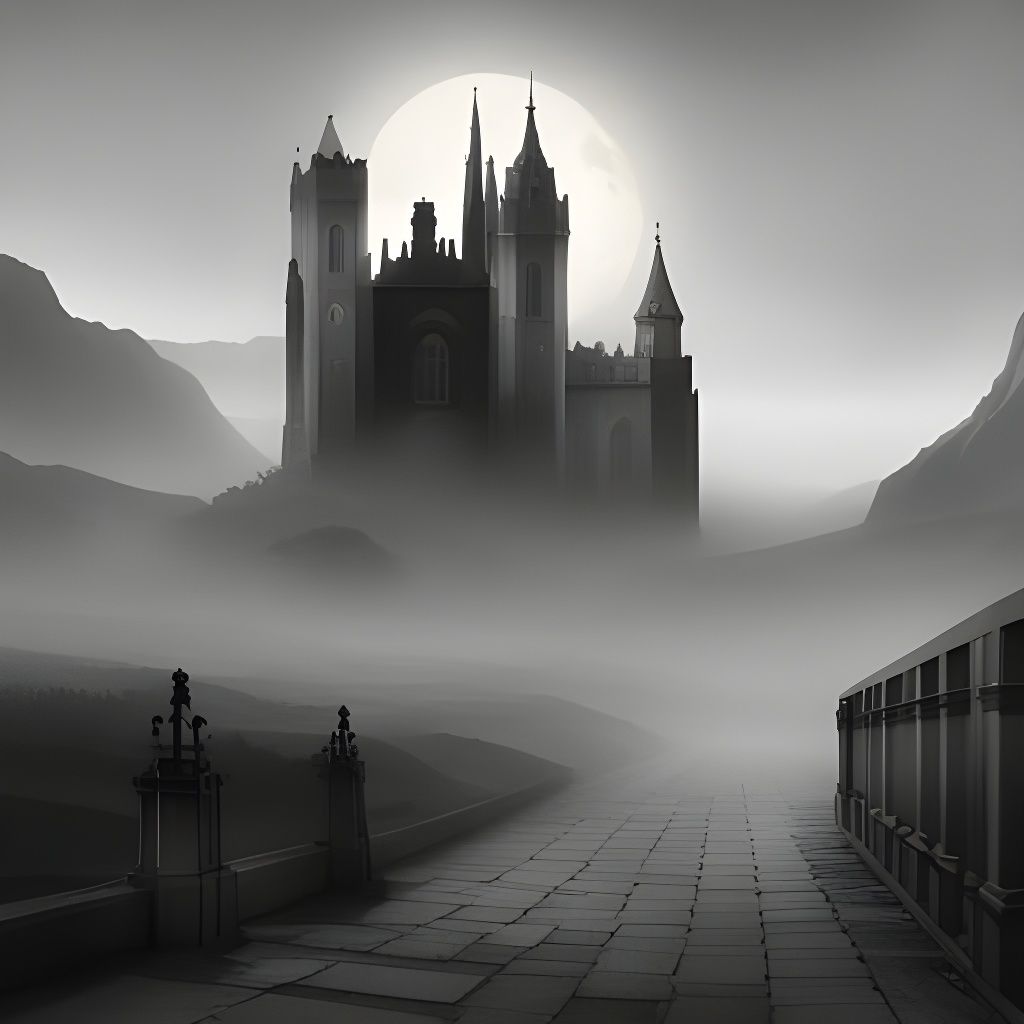The image is a black-and-white, gothic-inspired fan art or computer-generated drawing featuring a foreboding castle set in a foggy, mountainous landscape. The scene is dominated by a stone-tiled walkway that leads toward the imposing structure. On the right side of the path, there's a stone pillared wall or a fence made of concrete and metal that extends a short distance before being enveloped by the fog. The walkway itself is uneven, with antique-looking posts or small stone pillars lining a curb on the left side. Beyond this boundary, the ground appears hilly and grassy. Tall mountains rise on either side of the horizon, shrouded in thick fog that obscures parts of the middle of the image. A lone tree's top is visible through the mist. The castle, which is tall, gray, and intensely gothic with pointed steeples and windows, looms in the distance. Directly behind the castle, the moon shines brightly against the gray sky, partially hidden by one of the castle's steeples. The entire scene exudes a gloomy and eerie atmosphere, with varying shades of gray and black enhancing its dark, medieval aesthetic.